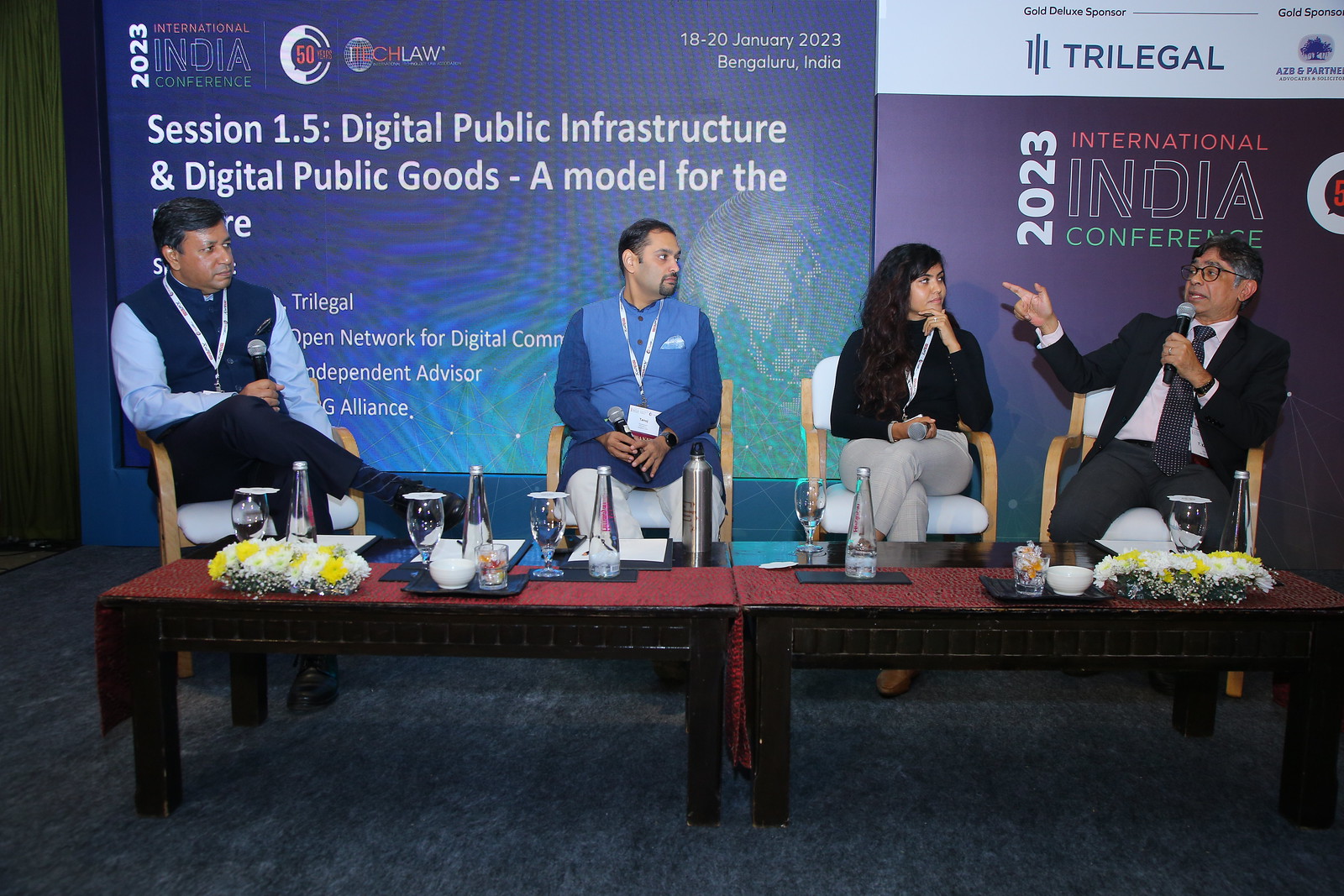In this detailed image, four individuals are seated at a series of long, low tables arranged across a room with carpet flooring. They appear to be engaged in a conversation, with one person holding a microphone. The tables in front of them are adorned with an assortment of objects including glasses, cups, plates, napkins, and small flower arrangements. Behind them, a large sign reads "2023 International India Conference" and "Session 1.5, Digital Public Infrastructure and Digital Public Goods." The full text of the sign is partially obscured. The color palette of the scene comprises various shades including gray, black, brown, red, white, yellow, blue, and green. This indoor setting is part of a conference, and the seating arrangement suggests a panel discussion or a similar event focused on digital public infrastructure.